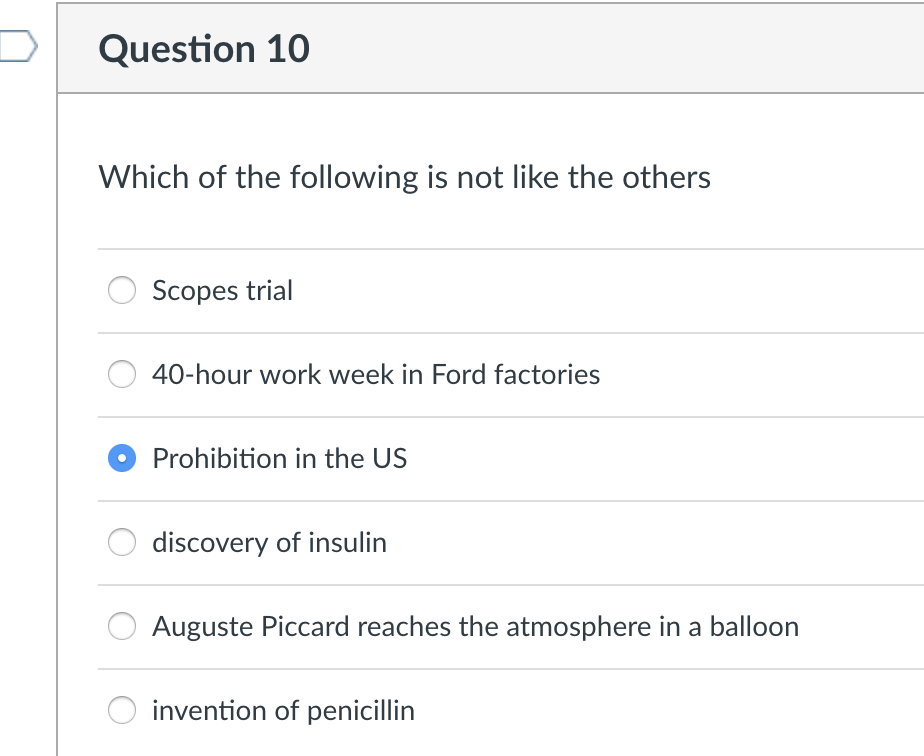The image depicts a question from a test or quiz, specifically labeled as "Question 10," with a structured layout that invites the participant to select an answer. The background features a large, rectangular box divided by lines into separate sections for clarity. 

The main query, "Which of the following is not like the others?" is prominently displayed at the top of the box. Below this question, five options are listed:

1. Scopes Trial
2. 40-hour work week in Ford factories
3. Prohibition in the US
4. Discovery of insulin
5. August Picard reaches the atmosphere in a balloon
6. Invention of penicillin

Each option has a circle next to it, intended for the participant to mark their selection. The specific choice "Prohibition in the US" is filled in with blue, indicating it's the selected answer.

In the top left corner of the image, there is a small bookmark symbol, suggesting that this question might be marked for review or importance. The background of the image is predominantly white, making the text and symbols stand out clearly.